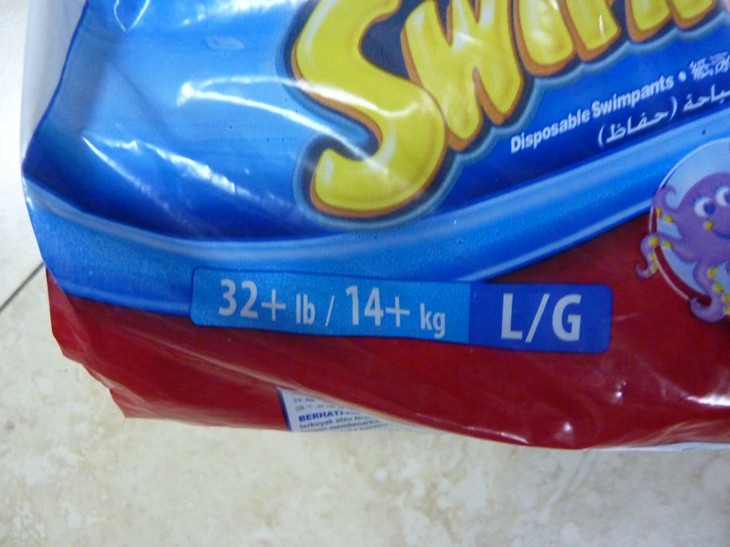The image depicts a package with a blue gradient top and a red bottom, commonly found on a marble stone surface. The upper blue section features yellow puffy lettering with only the letters "SW" partially readable. Directly beneath this, in white text, it reads "disposable swim pants." Below this text area is a light blue box displaying "32+ pounds / 14+ kg," adjacent to a darker blue box marked "L/G." To the right of these boxes, encircled in light blue, is an illustration of a purple octopus, with its right side cut off. Additional text in a foreign language, likely Chinese, is also present. The entire package appears to be made of plastic, resembling the material used for diaper packaging.